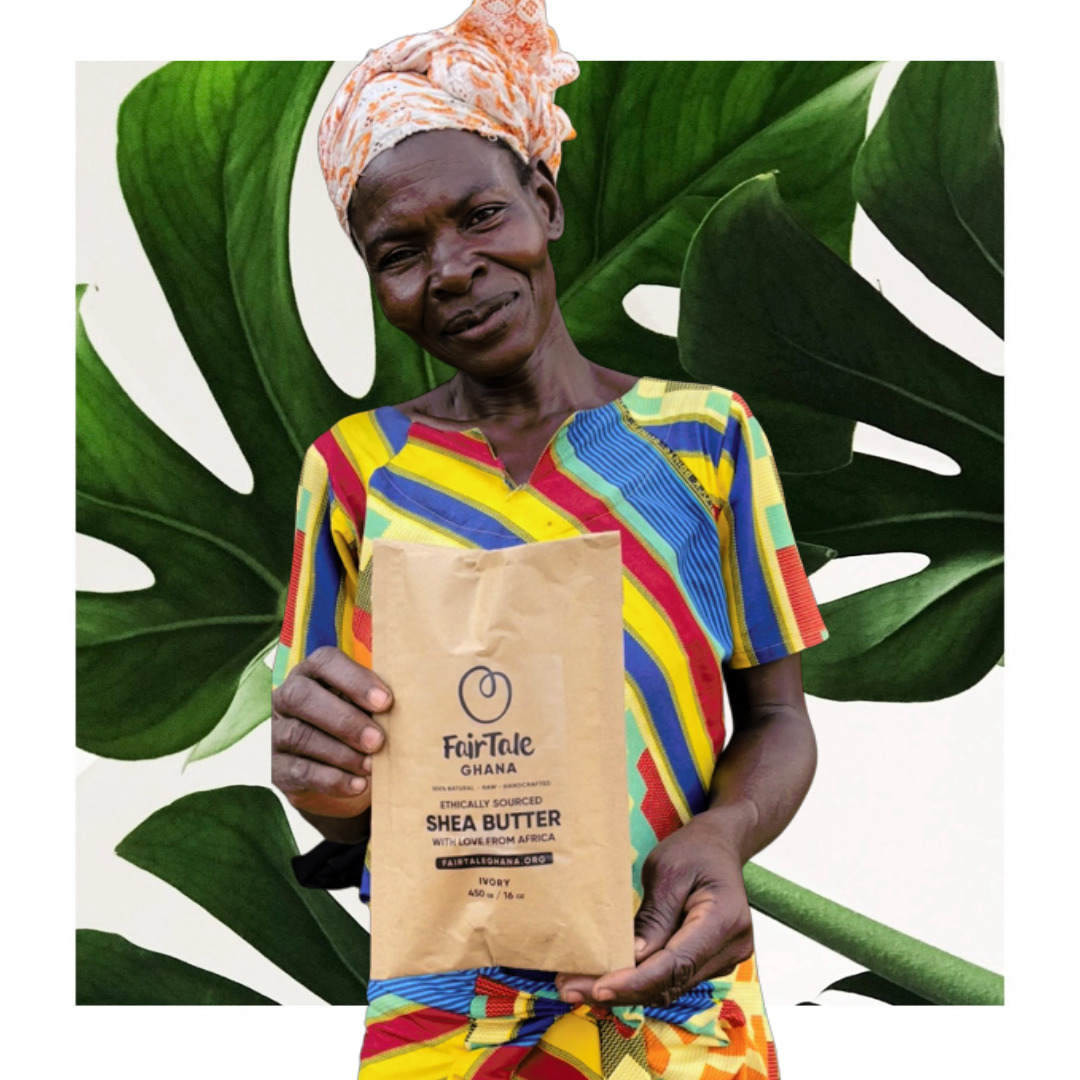A vibrant daytime photograph captures a dark-skinned woman in her late 40s to 60s, dressed in traditional African attire, posing outdoors against a white wall decorated with detailed green leafy vegetation. She wears a red, orange, and white cloth hat that is bunched to the right side of her head. Her multicolored striped shirt prominently features shades of yellow, red, blue, green, and light yellow, accented with splotches of orange near its base. She smiles warmly, her head slightly tilted, while holding a brown paper bag emblazoned with the text: "Fair Tail, Ghana, ethically sourced shea butter, with love from Africa," and in smaller letters, "Ivory 400, 16 count." Additionally, the packaging includes a ".org" website address. The photograph beautifully captures her colorful attire and the vividly detailed leafy backdrop.